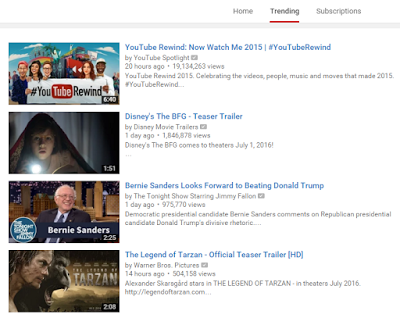This screenshot appears to be from an older version of the YouTube platform. At the very top, there are three primary options: Home, Trending, and Subscriptions. The Trending option is highlighted, displaying four trending videos.

1. **YouTube Rewind: Now Watch Me 2015 (#YouTubeRewind)**:
   - **Posted**: 20 hours ago
   - **Views**: Over 19 million
   - **Description**: This video celebrates the significant videos, people, music, and trends of 2015. 
   - **Context**: The high view count and the content's relevance suggest that the screenshot is from early 2016.

2. **Disney's The BFG – Teaser Trailer**:
   - **Posted**: 1 day ago
   - **Views**: Nearly 2 million
   - **Description**: This is the official teaser trailer for Disney’s adaptation of "The BFG".

3. **Bernie Sanders Looks Forward to Beating Donald Trump**:
   - **Posted**: 1 day ago
   - **Views**: 975,000
   - **Description**: Bernie Sanders discusses his optimism and strategies for the impending 2016 U.S. Presidential Election.

4. **The Legend of Tarzan – Official Teaser Trailer (HD)**:
   - **Description**: This is the high-definition, official teaser trailer for the movie "The Legend of Tarzan".

This image captures a nostalgic view of the YouTube interface and its trending section, reflecting popular content and political contexts from early 2016.